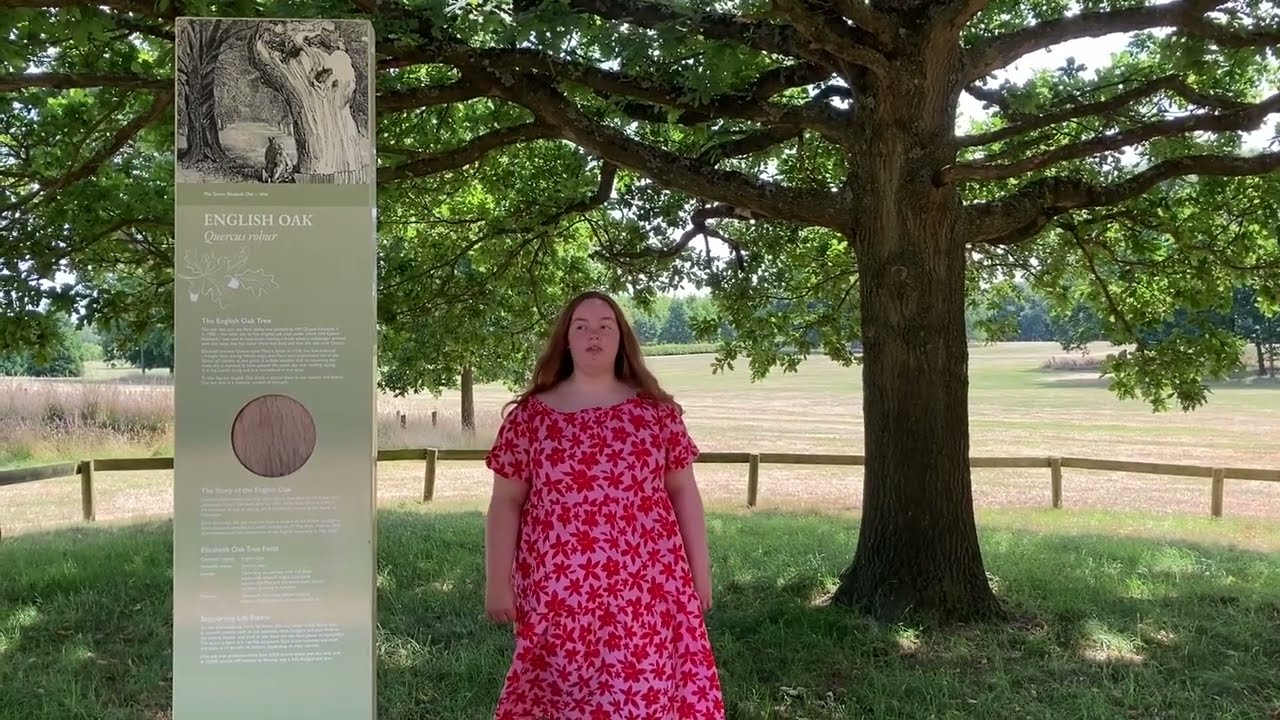In the photograph, there is a robust woman with long reddish-brown hair extending past her shoulders, standing in a sunlit park. She is wearing a striking muumuu adorned with red spots and pink and red floral patterns. Her gaze is off to her right, looking at something beyond the frame. To her left stands a memorial-like steel sign inscribed with "English Oak" and an undistinguishable text beneath it. Directly behind her is a tall English Oak tree, characterized by its many low-hanging branches and dense leafy canopy that creates a shaded area around the sign. Surrounding the grassy area where she stands is a single wooden railing fence, marking a clear boundary. The grass is mowed flat, except for a patch on the left where it appears taller. Through the thick branches, a bright sky is visible, though its details are washed out by the sunlight. The overall impression is of a tranquil, sun-drenched park setting.